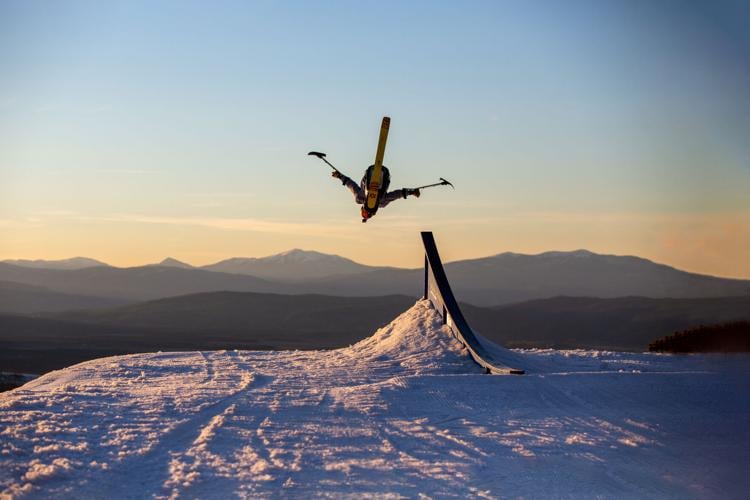This detailed photograph captures a high-flying skier performing an inverted aerial maneuver under a striking blue sky. The athlete is executing a loop with arms outstretched and his head pointing toward the snow-covered ground. He is suspended in mid-air above a ramp situated in the middle of the scene. The skier sports a vibrant yellow slalom ski and a red cap, adding bright splashes of color against the white snow and clear sky. The backdrop features majestic mountains and valleys, their peaks bathed in the soft, glowing light indicative of either early morning or late evening. The snow on the ground is marked with various trails, and the overall composition is framed in a landscape-oriented rectangle with a pronounced vignette effect in the corners, accentuating the action in the center. The vivid hues of white, red, yellow, sky blue, and shades of gray and black meld seamlessly to create a visually captivating and dynamic winter sports scene.